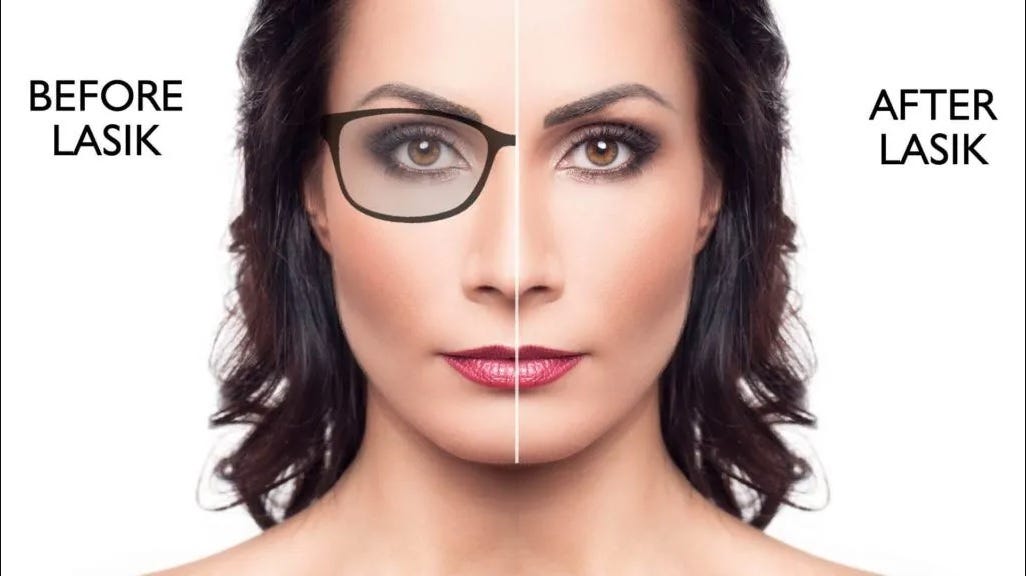The image is a promotional advertisement for LASIK surgery featuring a front-facing portrait of a woman. Her face is divided down the middle by a vertical white line, separating it into two halves: "Before LASIK" on the left and "After LASIK" on the right. The left side of her face, labeled "Before LASIK," depicts her wearing black-framed eyeglasses, which cast a slight shadow and give a more subdued impression. The right side, labeled "After LASIK," shows her without glasses, highlighting her enhanced appearance post-surgery. The woman has a short hairstyle that reaches her neck, dark brown hair, and a medium skin complexion. Her makeup is striking and well-defined, featuring smokey eyes, dark eyebrows, and red lipstick. The background of the image is white, and the picture showcases her from the neck up, with her bare shoulders faintly visible. The top of her head is cropped out. The advertisement clearly illustrates the visual benefits of LASIK surgery, emphasizing the woman's clearer, more vibrant look without glasses.